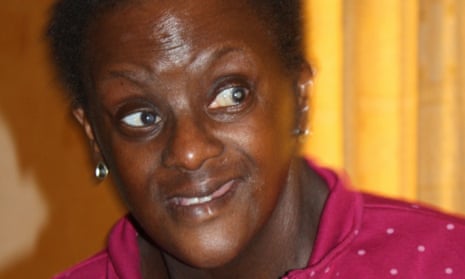A middle-aged African-American woman stands in front of a backdrop featuring a beige and yellow curtain on the right and a wall on the left. She has short, cropped hair and is wearing silver earrings. Her attire consists of a pink shirt adorned with white polka dots, which has a collar that's slightly askew. Illuminated by a camera flash, her eyes appear very white, and a glint highlights her nose while her forehead looks shiny. Her eyebrows are arched and her eyes are wide open, contributing to an expression that seems to combine curiosity with amusement and a hint of suspicion. Her lips are slightly parted in what could be a hesitant smile, partially revealing one of her cheeks. She gazes to the right side of the image, her face casting a shadow on the wall behind her. The colors in the photo include shades of pink, yellow, beige, and white.